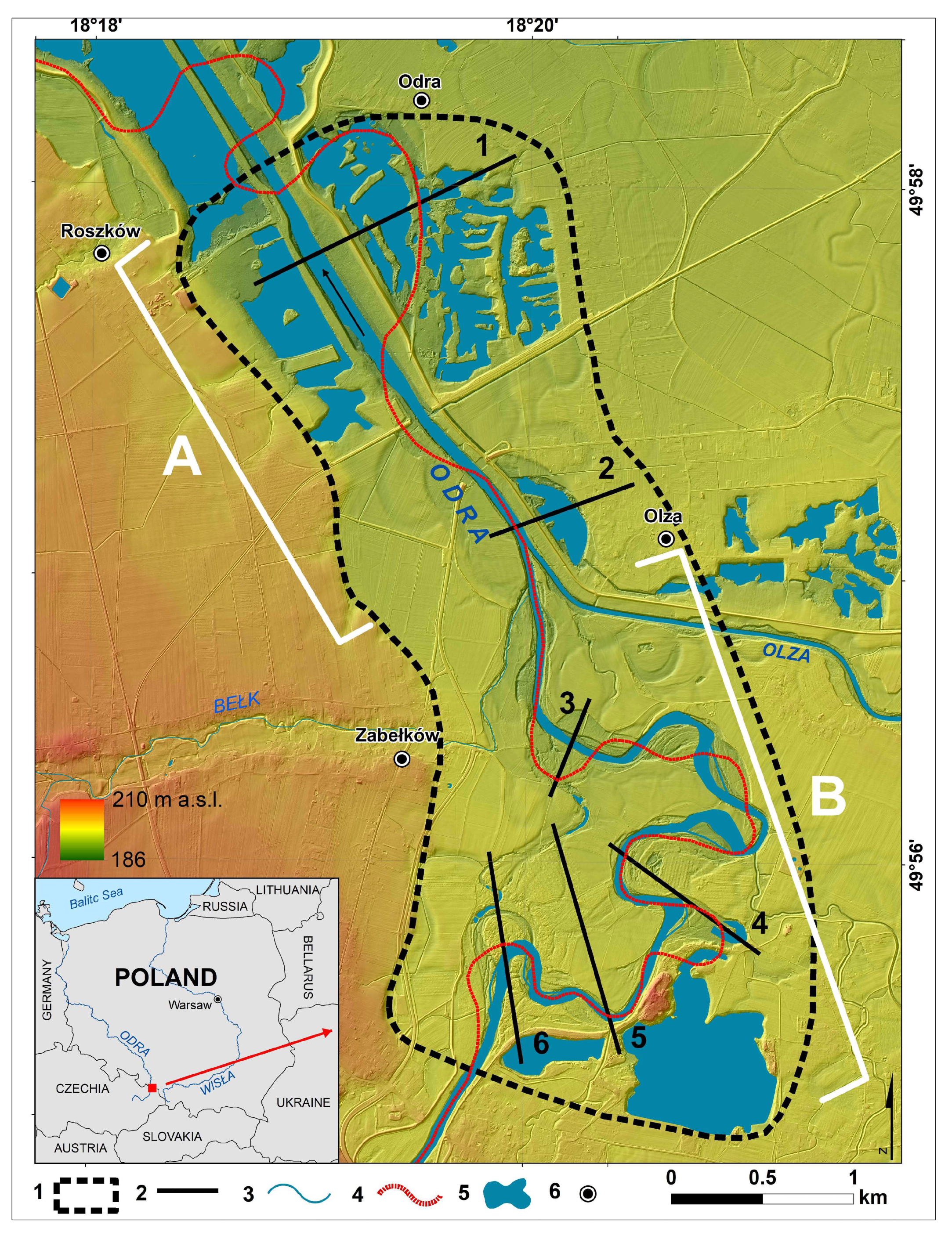The illustration is a detailed, drawn map featuring a bird's-eye view of the border region between Poland and Chechnya, with a specific emphasis on the Odra River and its surrounding areas. The map is rendered in green and brown colors, highlighting riverbanks and vegetation. A black outline demarcates the map's edges, indicating degrees and bearings. A key at the bottom of the image identifies various symbols, including a Tora square, solid lines, Kv lines, Kv dot-dashed lines, and river banks. The map indicates key locations such as Roskow, Zabolka, and Odra, presenting a region approximately 2 km wide and 15 km long. Additionally, a small inset map in the lower bottom left corner, marked with a red arrow, shows the position of the main map within a broader context of surrounding countries like Czechia, Slovakia, Ukraine, Belarus, and Russia. The text is in Polish, featuring names like Odra, Olza, and Roscoe. Notably, there is a scale bar ranging from 0 to 1 km, providing context for distances displayed on the map.